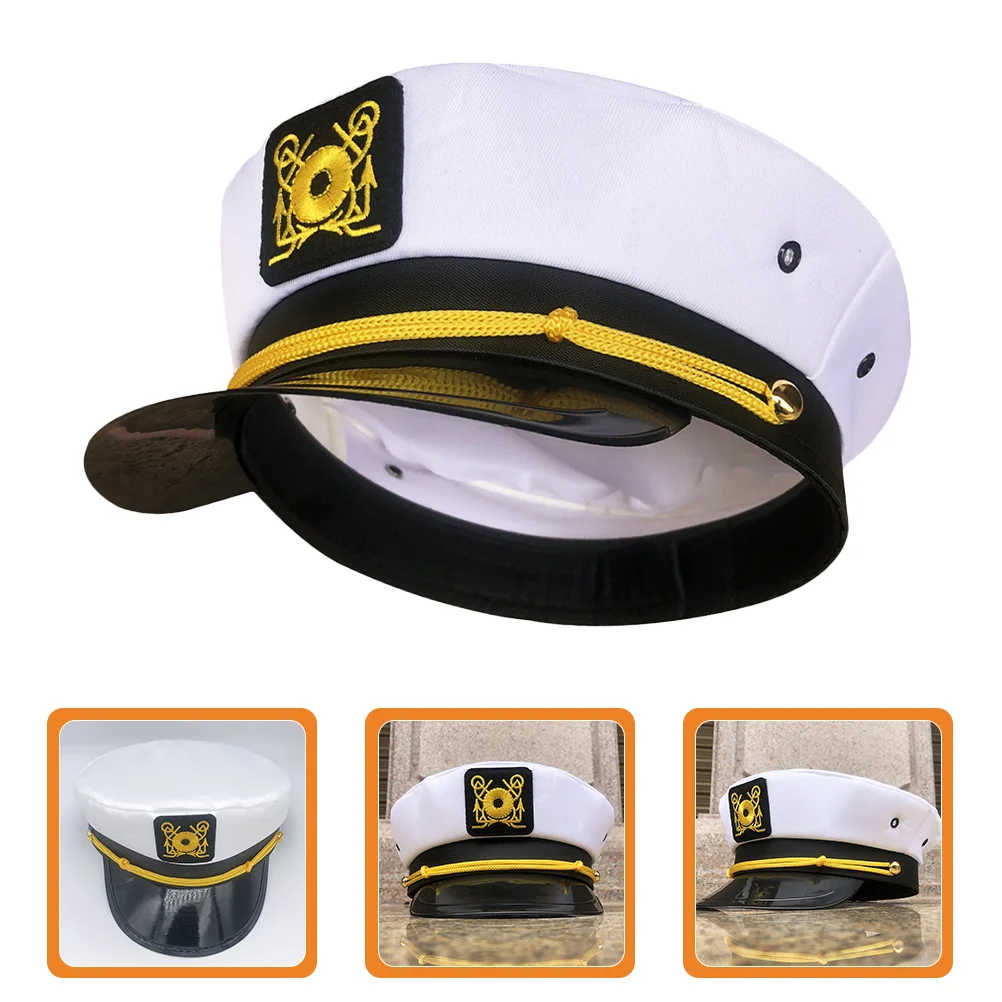This image features a sailor's cap displayed in four color photographs arranged in portrait orientation. The largest photograph at the top shows the cap from a side angle, with the brim pointing to the left, revealing some of the white lining inside. The cap is predominantly white with a black brim and features a gold rope affixed horizontally just above the brim. Prominently displayed on the front is a rounded black rectangular patch with intricate yellow embroidery consisting of a central circle bordered by arrows and circles.

Below the main image, there are three smaller photographs, each bordered by rounded orange squares, presenting different views of the hat. The leftmost image is a top-down view against a white background. The center image shows a direct frontal view of the cap placed on a beige marble surface. The rightmost photograph captures a side profile similar to the top image but without visible interior lining, also set on the beige marble surface. The images emphasize the details of the cap, focusing on its textures, colors (yellow, black, and white), and the settings, incorporating elements of photographic realism and product photography.